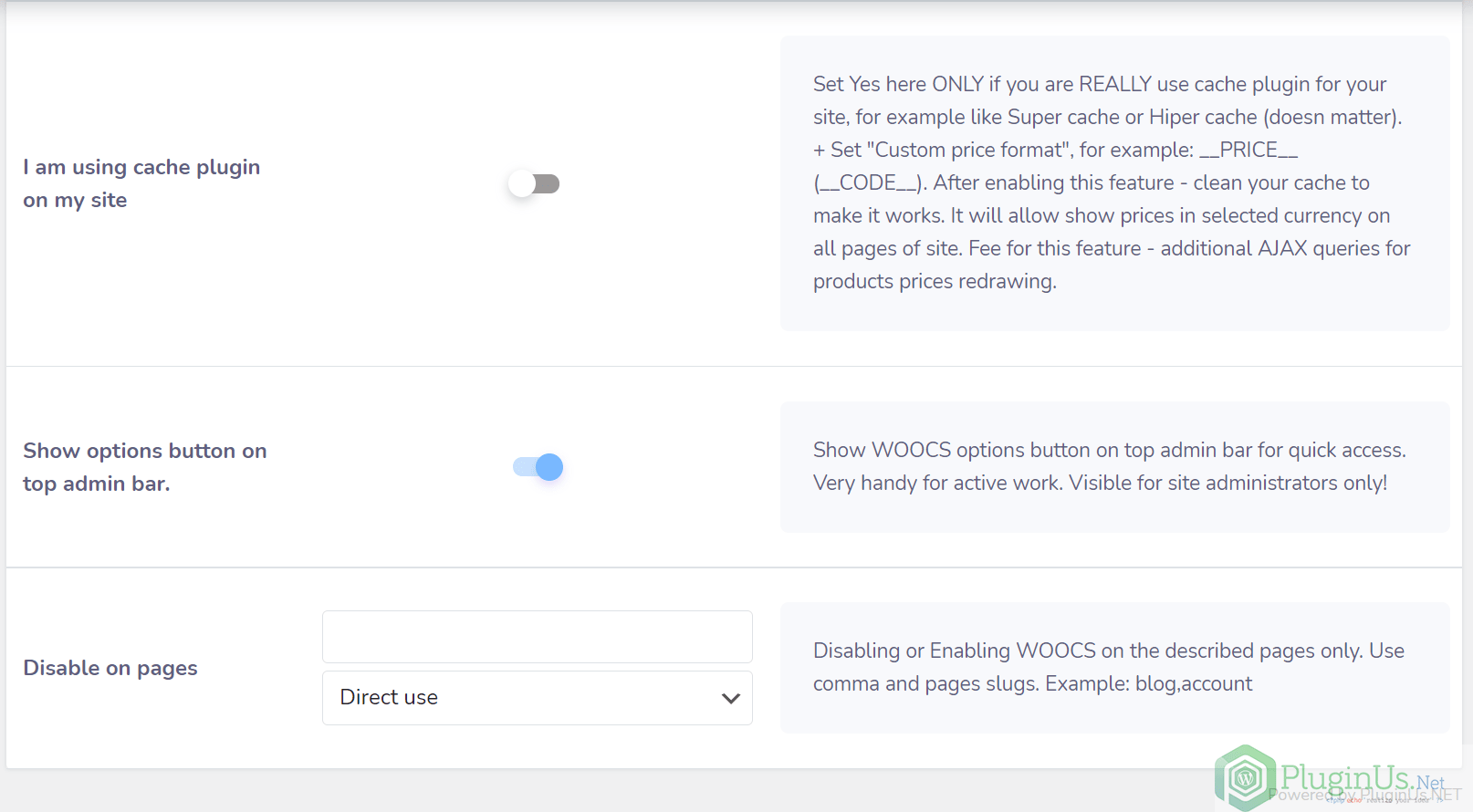**Image Description: Cache Plug-in Configuration Interface**

The image showcases a configuration interface for a website cache plug-in. The main section of the interface is presented on a white screen bordered by a thin gray line. 

- **Upper Left Section:** Here, a label reads "I am using cache plug-in on my site." Below this label, there is a toggle switch set to the off position.
  
- **Upper Right Section:** A descriptive note states, "Set 'Yes' here only if you are really using cache plug-ins for your site, such as Super Cache or Hyper Cache. Additionally, set a custom price format in parentheses, e.g., '_price_' or '_code_'. After enabling this feature, clean your cache to make it work. This setup will show prices in the selected currency on all pages of the site, but it may also incur additional AJAX queries for product price retrieval."

- **Middle Left Section:** There is another option labeled "Show button options on top admin bar," which is toggled on.

- **Middle Right Section:** An elaboration explains, "Show WOOCS option button on the top of the admin bar for quick access. Very handy for active work. Visible for site administrators only."

- **Bottom Left Section:** The option "Disable on pages" is visible with an associated data field and a dropdown menu labeled "Direct use." It indicates that this setting disables or enables WOOCS on the specified pages only. The user is instructed to use commas and page slugs, for example, 'bot.account.'

- **Bottom of the Interface:** The footer includes a reference to "plugins.net."

This structured and detailed caption gives a comprehensive overview of the various settings and instructions provided in the interface.